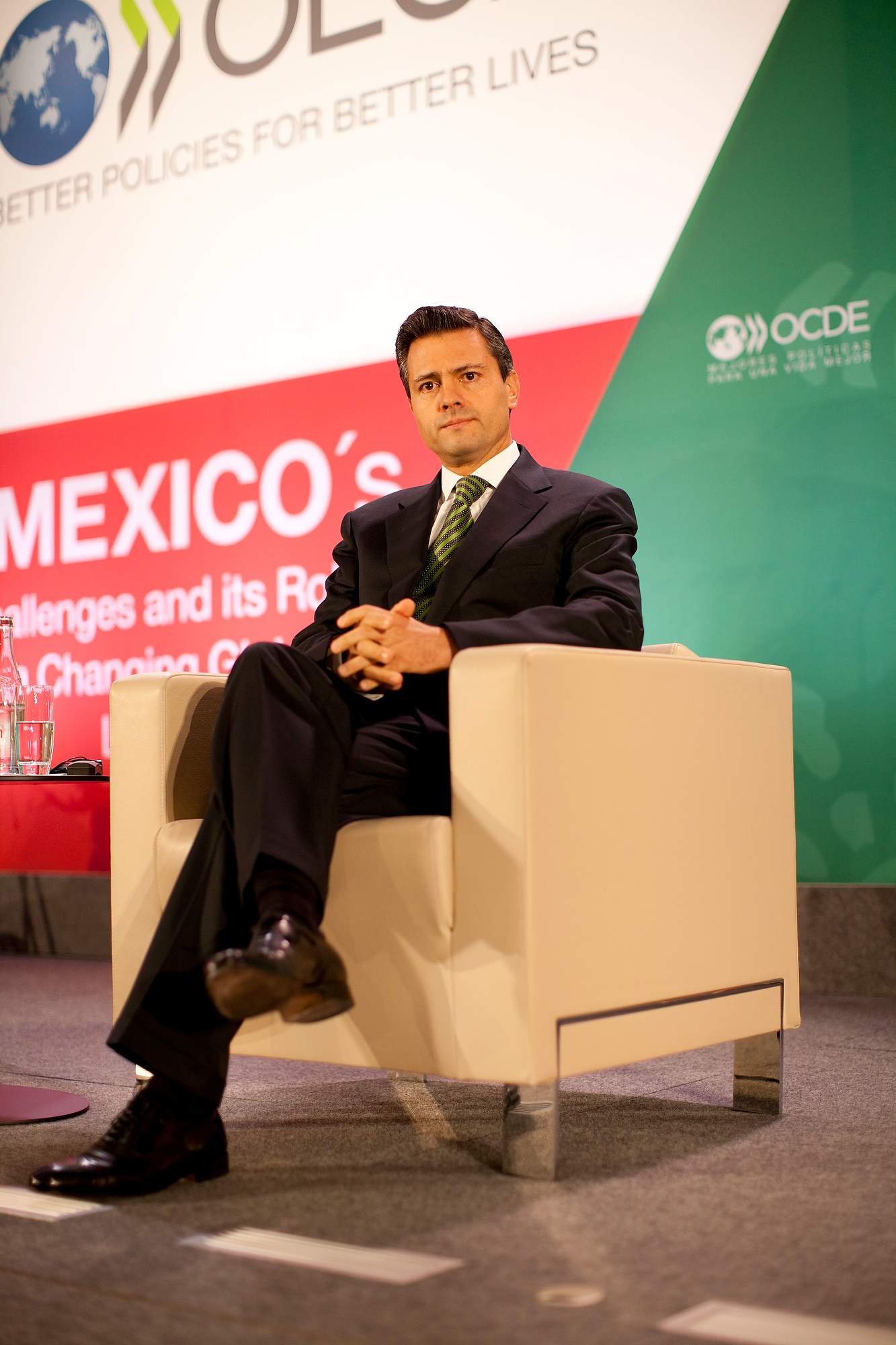In the photograph, a man, presumably a politician or spokesperson, sits on a stage in a squared, beige upholstered chair with tall sides and triangular metal legs. His polished black shoes with brown soles peek from under his black dress pants as he rests his right leg over his left knee. With his fingers intertwined in his lap, the man appears composed yet focused, wearing a black business coat over a white button-up shirt and a green and black striped tie. His black hair is neatly styled to a point, and his dark, clean-shaven face maintains a neutral expression as he gazes at the camera. To his right is a small table holding a glass of water and a water bottle. A backdrop behind him features a banner in red, white, and green that reads "Mexico's Challenges: Better Policies for Better Lives," with an image of the planet Earth and the acronym OCDE.